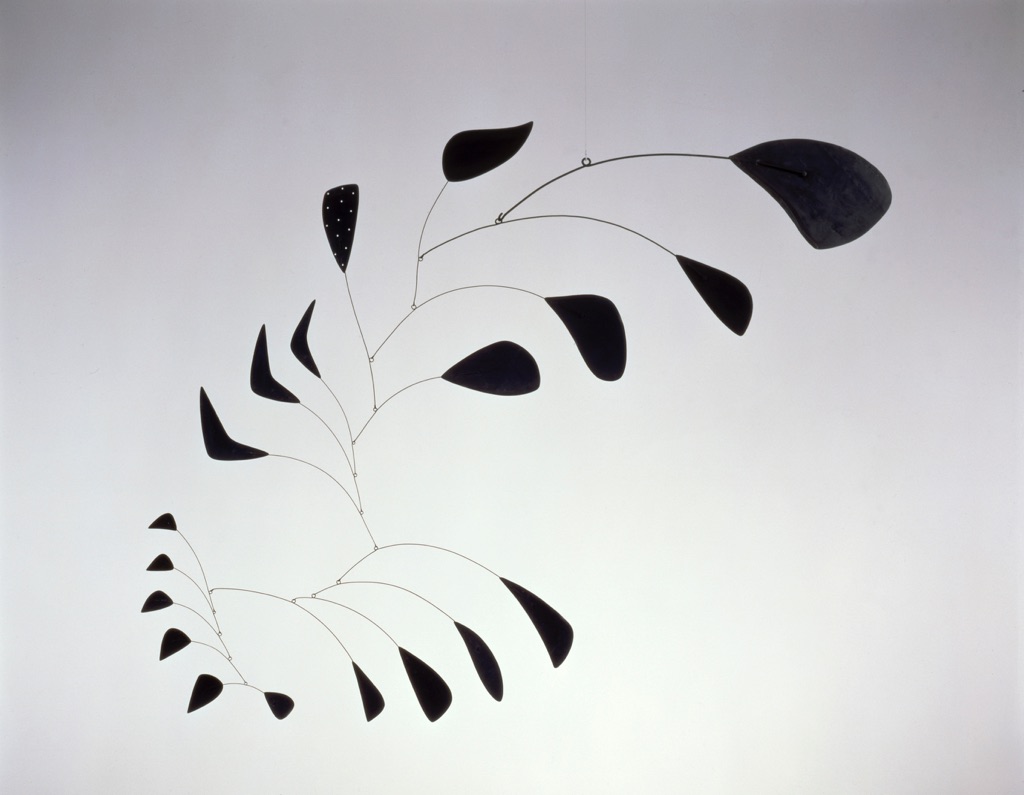The image is a photograph of an abstract painting depicting a plant-like mobile or sculpture. The background is predominantly white with a gradient effect, transitioning to dark gray in the top two corners and light gray in the bottom two corners. A thin wire hangs from the center of the image, attached to the sculpture by a small loop. The sculpture consists of multiple black, thin, wire-like stems that extend from a central point and become progressively smaller from right to left. Each stem ends in a solid black leaf-shaped object. The stems are interconnected by loops located either at their centers or bottoms. The overall composition has a branching effect, with leaves resembling black blobs or boomerangs, contributing to the intricate, abstract nature of the artwork. The image contains no dates, signatures, words, numbers, or people.